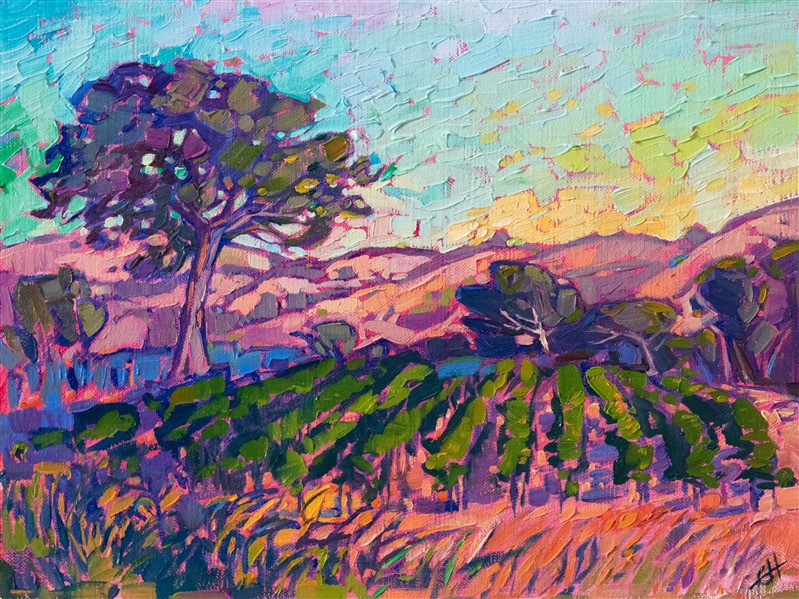The image is a detailed oil painting on canvas, characterized by its visible brushstrokes and layered texture. It depicts an outdoor scene, most likely a vineyard or farmland. Dominating the left side is a large tree with green leaves and a sturdy brown trunk, and a smaller tree stands nearby. The right side showcases neatly arranged rows of green vines or crops. The foreground features grassy areas interspersed with brown patches, suggesting dirt. The background reveals rolling hills painted in pink and purple hues. The sky above transitions from a light blue to a yellowish tint, indicating a possible sunrise or sunset. The overall color palette includes pastels and cool tones like blues, greens, and purples, reinforcing an impressionistic style. Initials "CH" can be seen in the bottom right corner of the painting.